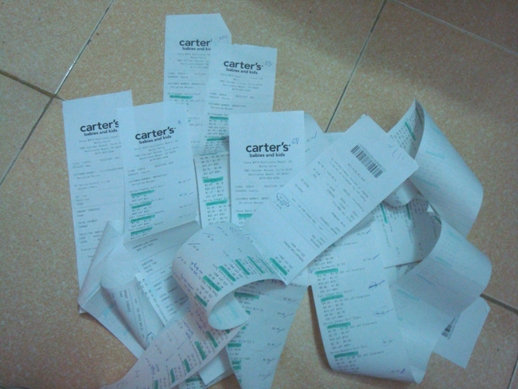The photograph is a detailed color image depicting a disorganized pile of at least a dozen long, white receipts from Carter's store scattered on a bathroom floor. Each receipt is marked with the store's name in black at the top, with additional black text outlining individual purchases. Various amounts on the receipts are circled or highlighted with green marker, indicating a review or verification process. The receipts are tangled and curled, lying across large, square tiles that are a brownish-orange hue. The tiles feature visible cracks filled with dirt and debris, further contributing to the apparent clutter.